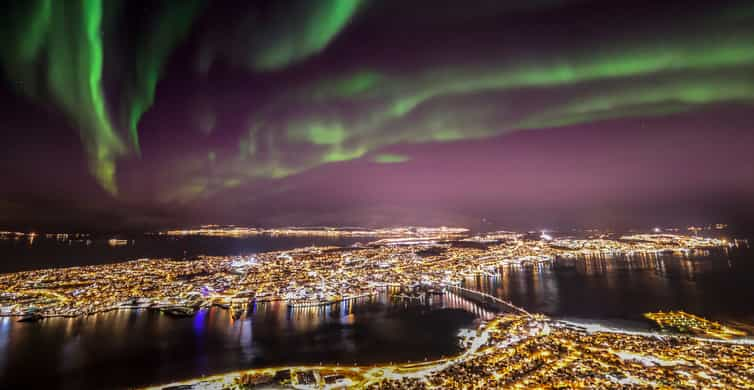The image captures a breathtaking, panoramic night view from the observation platform at the top of the Fjellheisen cable car in Tromsø, Norway. The iconic Tromsø Bridge arches gracefully over the water, connecting the mainland to the island area of the city, which is illuminated with bright, golden lights that cast a vibrant glow across the landscape. The harbor and cityscape spread out below are bathed in this luminescent aura, further highlighting the scenic beauty of Tromsø.

Dominating the upper half of the image, the northern lights dance across the dark sky in a stunning display of green, greenish-gray, and pink hues, blending with the purple tones of the twilight atmosphere. This ethereal light show provides a striking contrast to the city’s artificial lights and the tranquil expanse of water that divides the city. The overall clarity and vividness of the photograph showcase the radiant, colorful essence of Tromsø by night, making this image a captivating testament to the Arctic city's natural and urban splendor.